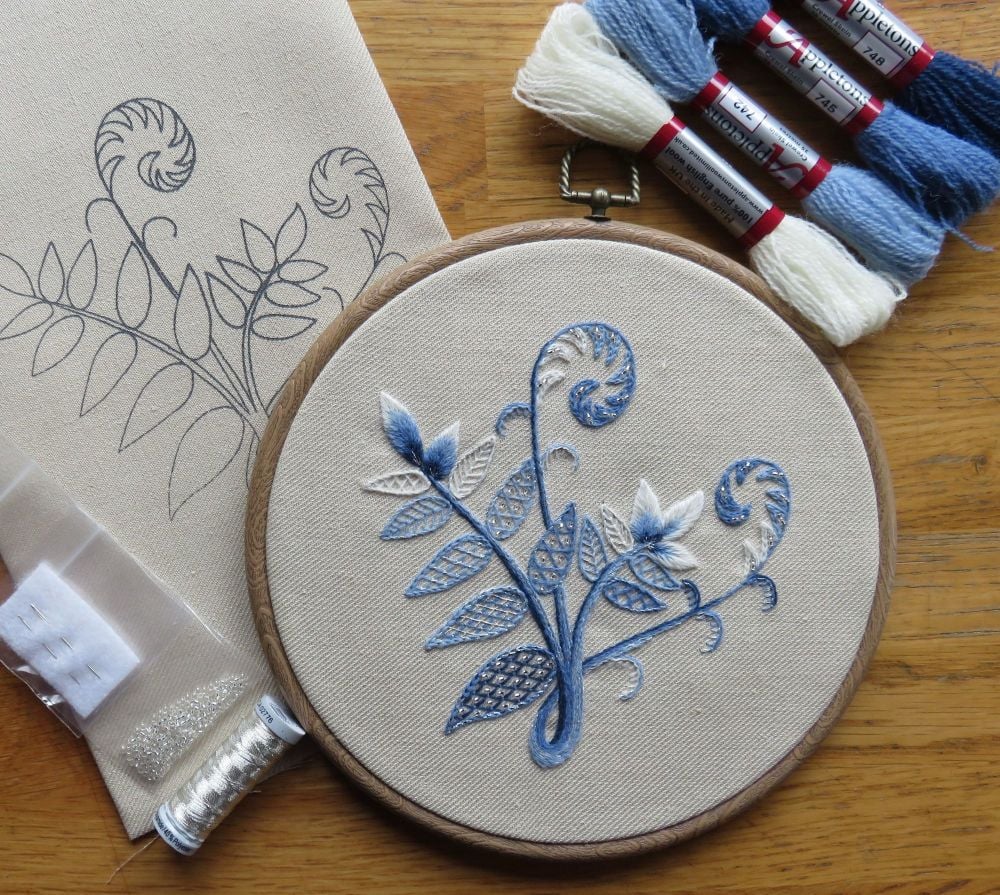This photo shows an embroidery kit, meticulously laid out on a wooden surface. Central to the image is an embroidery hoop containing a piece of off-white, light beige fabric with an intricate design already embroidered on it. The design features a plant with various leaves and curled stems, interspersed with flower petals, all stitched in shades of blue and white.

To the left of the hoop, there is a folded piece of cloth with the same pattern sketched in black marker, serving as a stencil for the embroidery design. In the top right corner, we see four spools of thread in a gradient of colors: dark blue, medium blue, light blue, and white.

Additionally, a small plastic bag with a piece of felt holds a couple of needles and very tiny, clear beads along with metallic silver thread. The kit comprehensively includes all the essentials needed for creating the embroidered plant with leaf and flower patterns, emphasizing the various shades of blue and the detailed artistry involved.